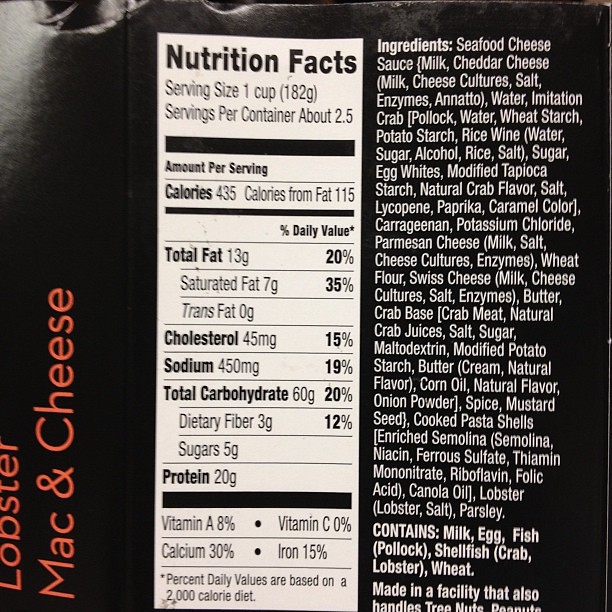This image showcases the Nutrition Facts label on the back of a package of lobster mac and cheese. On the left side of the image, the product name "Lobster Mac and Cheese" is displayed vertically in bold orange letters against a black background. The same black background is used for the Nutrition Facts label, which is presented in white font.

The label starts with a comprehensive list of ingredients used in the dish. Below the ingredient list, a warning is printed in bold lettering indicating that the product contains milk, egg, fish (pollock), shellfish (crab, lobster), and wheat. It also notes that the product is made in a facility that handles tree nuts and peanuts.

Adjacent to the ingredient list, a white rectangular box encloses the detailed Nutrition Facts. The text within this box is in black font, providing essential nutritional information. The serving size is specified as one cup, with approximately 2.5 servings per container. Each serving contains 435 calories, with 115 calories derived from fat.

The label continues to delineate the percent daily values of various nutrients: total fats, saturated fat, trans fat, cholesterol, sodium, total carbohydrates, dietary fiber, sugars, protein, vitamin A, calcium, and more. Key nutritional highlights include 13 grams of total fat, 45 milligrams of cholesterol, 450 milligrams of sodium, 60 grams of total carbohydrates, and 20 grams of protein per serving.